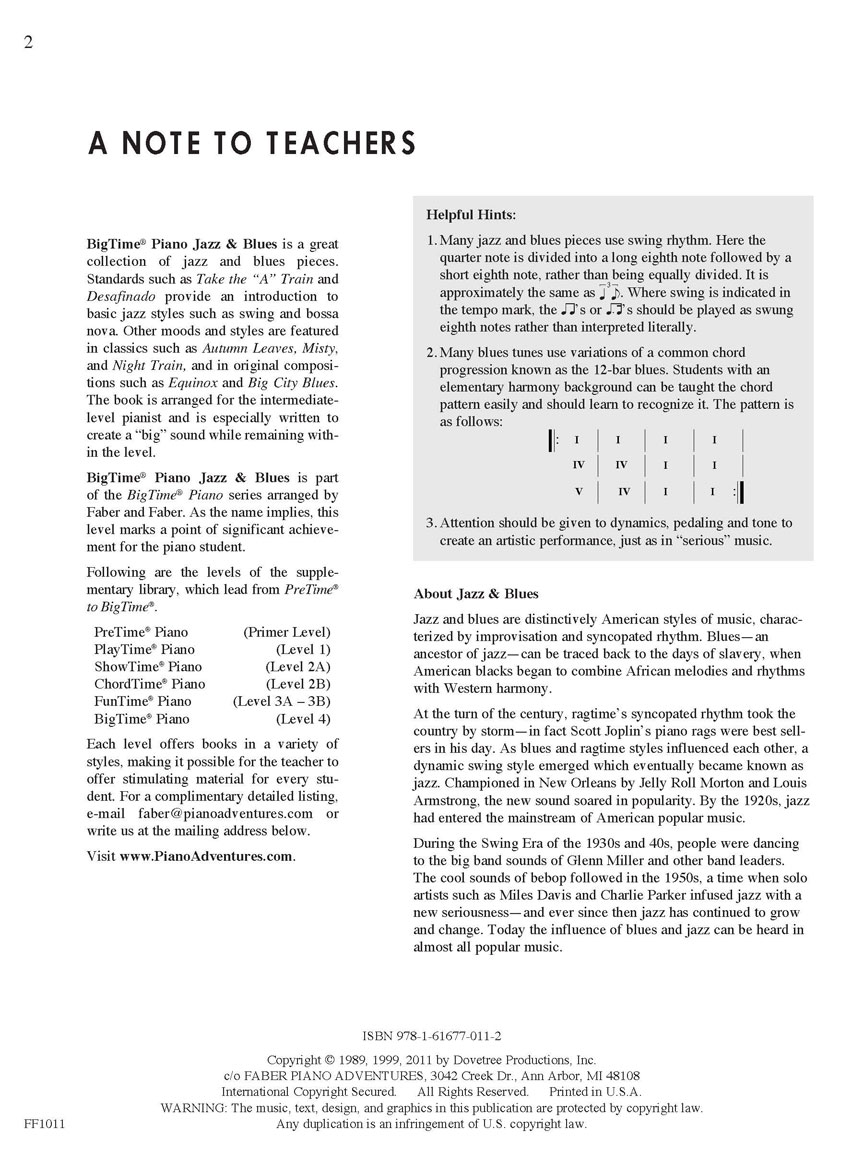This image depicts the second page from a music instruction book titled "Big-Time Piano Jazz and Blues," which features a note to teachers at the top. The printed black and white page introduces the distinct American music styles of jazz and blues, highlighting their historical significance and characteristic harmonies. The text, though small and somewhat challenging to read, includes several paragraphs with helpful hints and guidelines for teaching beginner to more experienced piano students. It also features a table outlining these helpful hints. The link www.pianoadventures.com is provided for additional resources. At the bottom of the page, there is extensive legal text, including copyright information dated 1982-1999 and 2011, ISBN details, and it notes that the book was printed in the USA.